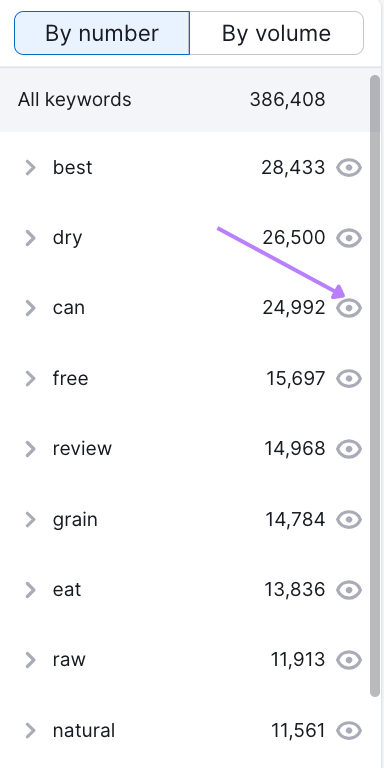This image is a screen capture from a mobile device, oriented in a vertical format and about twice as tall as it is wide. The capture includes the entire screen, except for the top and bottom control panels. The background of the screen is white, featuring black text.

At the top of the screen, there are two buttons. The button on the left, highlighted in blue, is labeled "By Number," while the button on the right, not highlighted and in white, reads "By Volume." Just below these buttons, a light gray banner stretches across the screen with the text "All Keywords 386,408."

Below the banner, the screen is divided into two side-by-side columns displaying a list of keywords. Each keyword appears on the left, accompanied by numerical values on the right. There are nine keywords listed from top to bottom: "best," "dry," "can," "free," "review," "grain," "eat," "raw," and "natural." The numbers next to these keywords range from approximately 11,000 to 28,000.

To the right of each number is a gray eye icon outline, representing visibility. A purple arrow is prominently featured, pointing downward and slightly to the right at an angle, specifically targeting the third eye icon from the top, which is next to the keyword "can."